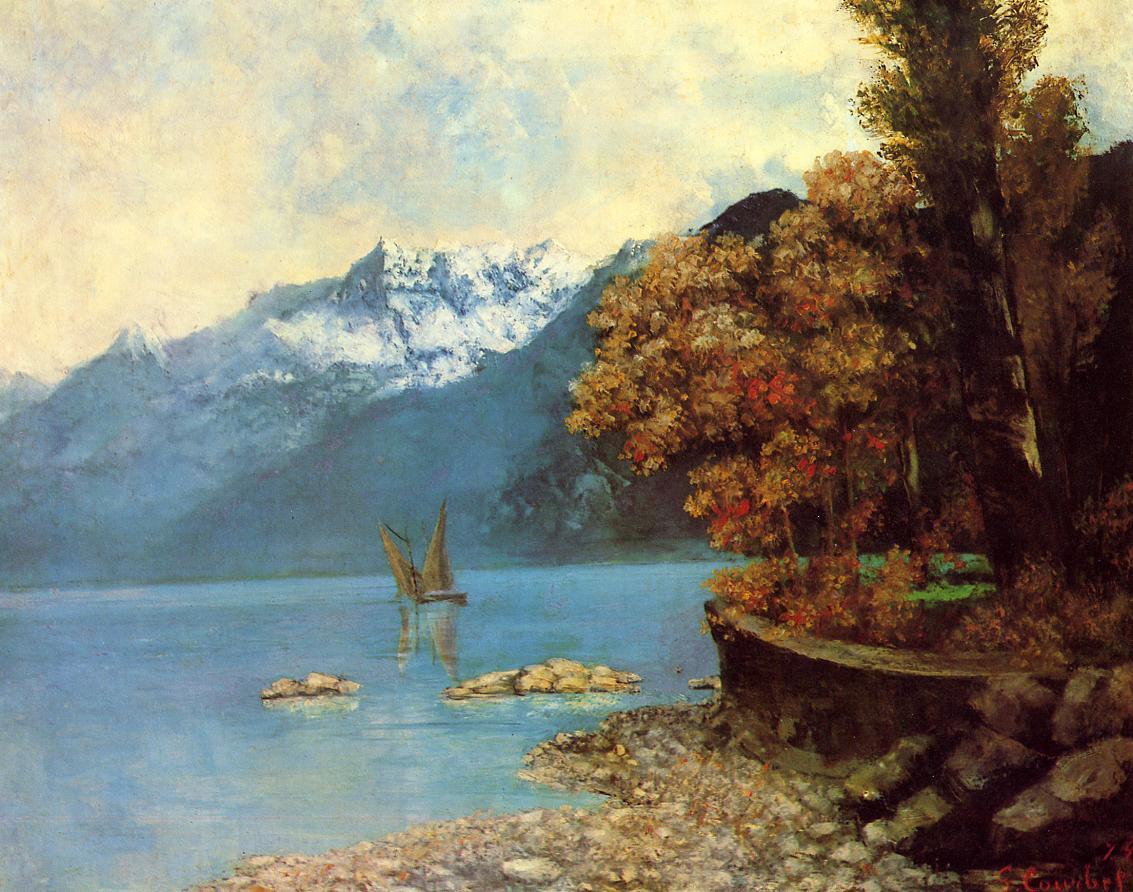This detailed painting portrays a tranquil outdoor landscape with majestic snow-covered mountains on the left, their white peaks and blue highlights towering against a lightly yellow-tinged sky adorned with fluffy white clouds. To the right is a vibrant, autumn-colored tree with red, orange, and gold leaves, situated within a fenced enclosure that contains grey rocks and foliage. Dominating the scene, a serene, turquoise-colored body of water, reflecting a sailboat with two sails, lies at the center. Surrounding the water are rocky structures that emerge intermittently. The mountains transition from a bright snow-topped blue to a darker, muted gray-blue as they fade into the distance. This bucolic scene further includes a rocky shore near the lower right corner, and the painter’s barely legible signature graces the bottom right of the artwork. The palette features a rich blend of colors: black, white, gray, various blues, tan, brown, orange, red, yellow, and a hint of green, capturing the essence of a peaceful, autumnal day.